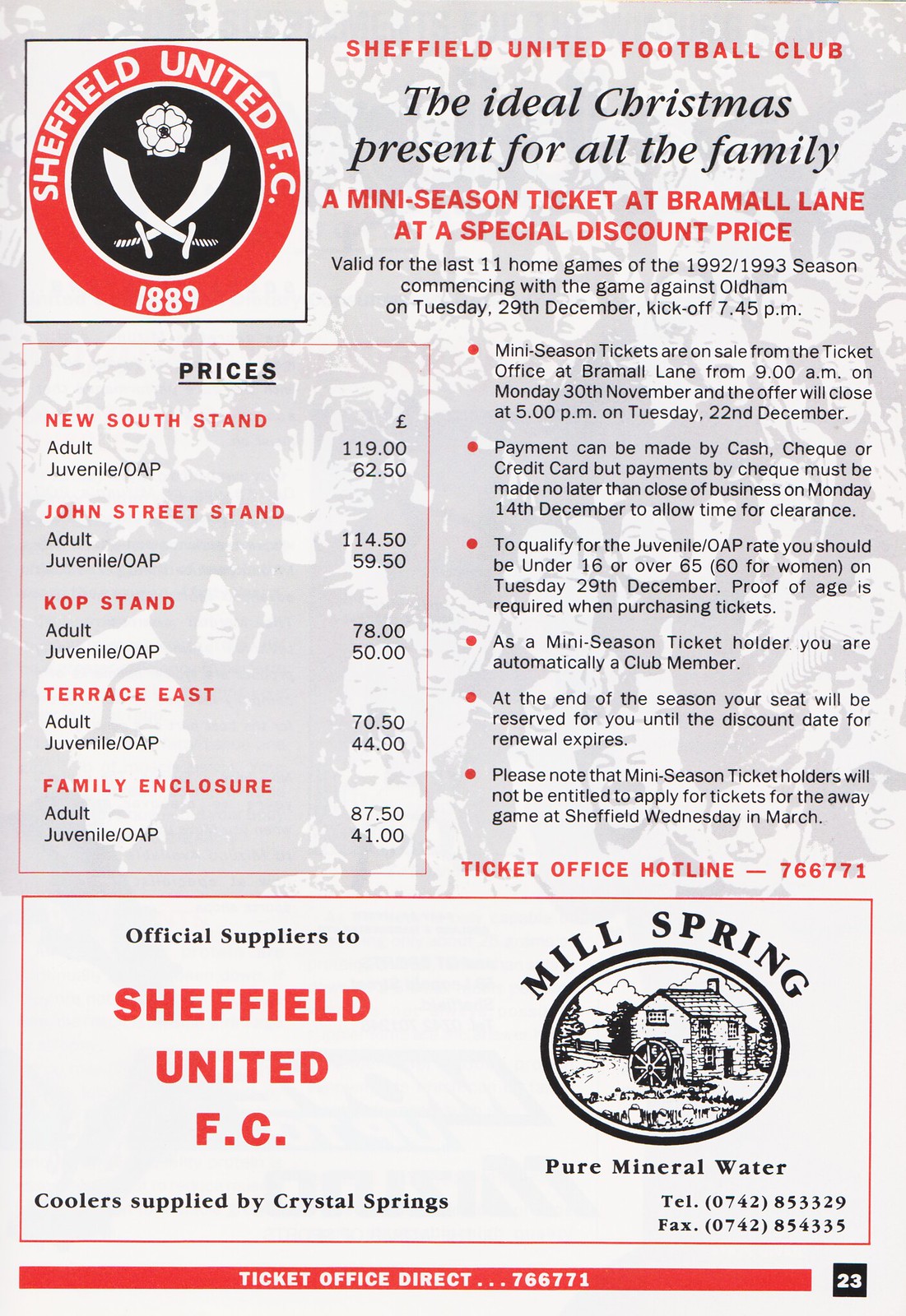This is a color advertisement for Sheffield United Football Club. In the top left corner, the club’s logo is prominently displayed, featuring the text "Sheffield United FC, 1889" and two crossed swords. The header reads in red, "Sheffield United Football Club: A Mini-Season Ticket at Bramall Lane at a Special Discount Price." Below that, in black text, it proclaims, "The Ideal Christmas Present for All the Family." It details that the mini-season ticket is valid for the last 11 home games of the 1992-1993 season, starting with the game against Oldham on Tuesday, 29th December, with a kickoff at 7:45 pm.

On the left side of the flyer, there is a rectangular box listing ticket prices for various stands: New South Stand (Adult £119, Juvenile £62.50), John Street Stand (Adult £114.50, Juvenile £59.50), KOP Stand (Adult £78, Juvenile £50), Terrace East (Adult £70.50, Juvenile £44), and Family Enclosure (Adult £87.50, Juvenile £41). 

At the bottom, there's an advertisement for Mill Spring Pure Mineral Water, noting it as the official supplier to Sheffield United Football Club, with coolers provided by Crystal Springs. Lastly, the ticket office contact number is given as 788771, alongside a notation of "23" in the far right corner.